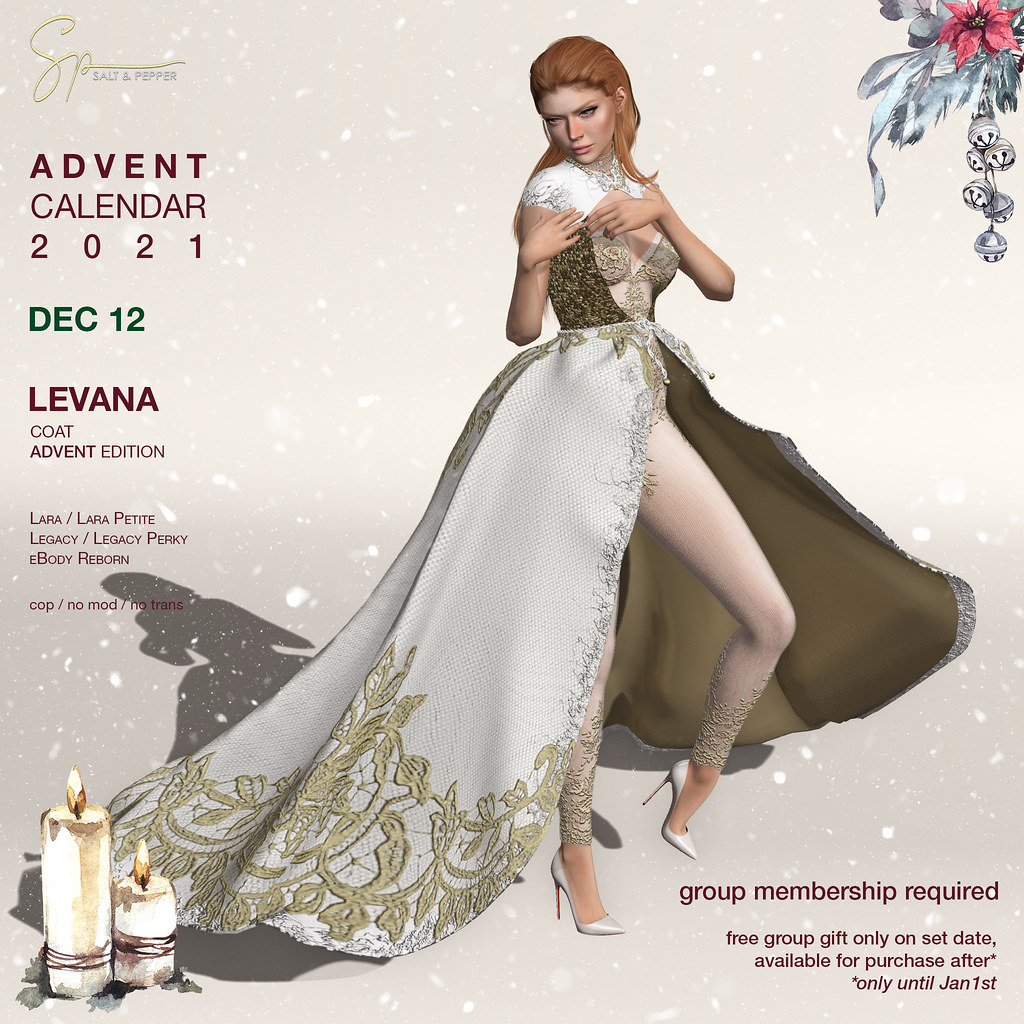In the image, which appears to be a digitally-rendered cover or advertisement for an advent calendar, a central focus is a 3D-rendered woman dressed in an elaborate outfit. The woman, a Caucasian female with long red hair, stands prominently in the center. She wears a white corset with gold trim and short sleeves, paired with white tights and high heels. Her flowing, open-front dress is white with golden leaf trim along the bottom edge and a tan interior.

The text on the left side of the image reads, "Salt and Pepper Advent Calendar 2021, December 12th, LaVanna Coat Advent Edition, Lara / Lara Petite, Legacy / Legacy Perky, eBody Reborn, Copy / No Mod / No Trans." Additionally, in the bottom right corner, it states, "Group membership required. Free group gift only on set date. Available for purchase after, only until January 1st."

The image also showcases two lit candles at the bottom left and some flowers in the top right, contributing to the festive and decorative feel, suggestive of use around Christmastime.